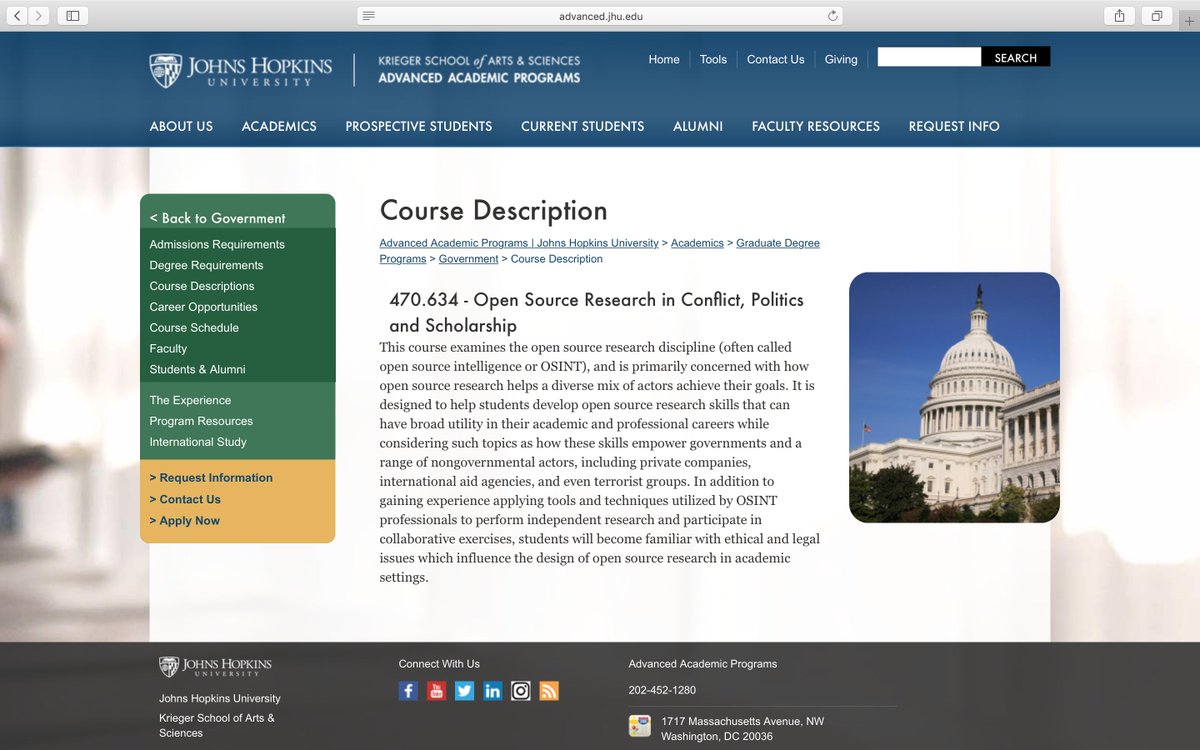The image captures a detailed view of a university course webpage on a browser, specifically the website for Johns Hopkins University Krieger School of Arts and Sciences Advanced Academic Programs, as indicated by the URL "advanced.jhu.edu" at the top.

The top banner of the website, displaying a blue background with white text, prominently features the institution's name and the school's division. Below the banner, a horizontal navigation menu is visible with options labeled Home, Tools, Contact Us, and Giving. Adjacent to this menu is a search bar, equipped with a large black button marked "Search."

Below this primary navigation, there is a second row of tabs for more specific navigation. The tabs read: About Us, Academics, Prospective Students, Current Students, Alumni, Faculty Resources, and Request Info. The webpage being viewed is dedicated to a specific course, with the heading "Course Description" followed by a breadcrumb trail providing context within the website's structure.

The course title in bold text reads "470.634 - Open Source Research and Conflicts, Politics, and Scholarship". There is a comprehensive course description beneath this heading. Accompanying the text, on the right side of the page, there is an image of an official building characterized by its grand dome, numerous pillars, surrounding trees, and a blue sky overhead.

On the left side of the page, a sidebar lists several links. This list includes the following: Back to Government, Admissions Requirements, Degree Requirements, Course Descriptions, Career Opportunities, Course Schedule, Faculty, Students and Alumni Experience, Program Resources, International Study, Request Information, Contact Us, and Apply Now.

The bottom of the webpage is designed with a dark grayish-brown banner, which features contact information, phone numbers, and additional information about the university.